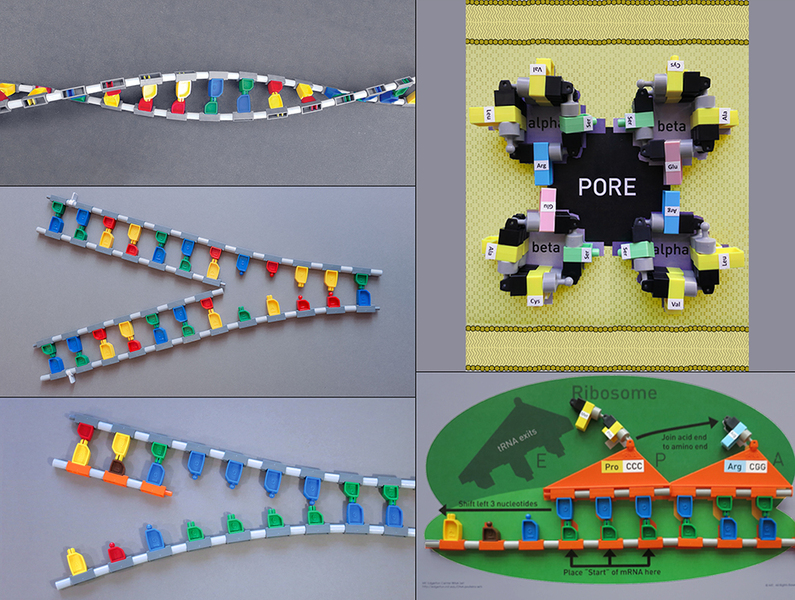The image showcases five distinct panels, each depicting elements related to DNA and molecular biology against a unified grey background. In the top left corner, there's an illustration of a typical multicolored DNA strand comprised of interlocking pieces in blue, red, and yellow. Below this, another panel shows two DNA strands splitting and merging back together, forming a Y shape, and further below, a similar image depicts a partially split DNA strand slightly rejoining at one end. On the top right, there's a detailed diagram labeled "PORE" at its center, surrounded by structural labels such as alpha and beta in each corner. This diagram appears to be held together by word blocks, emphasizing its functional components. Finally, in the bottom right, there's an image featuring a ribosome with various descriptive annotations. It shows detailed instructions including "IRNA exits," "ribosome," "join acid end to amino acid," and "place start of mRNA here." Each panel collectively illustrates various forms and configurations of DNA and related structures, offering an in-depth view of molecular interactions.